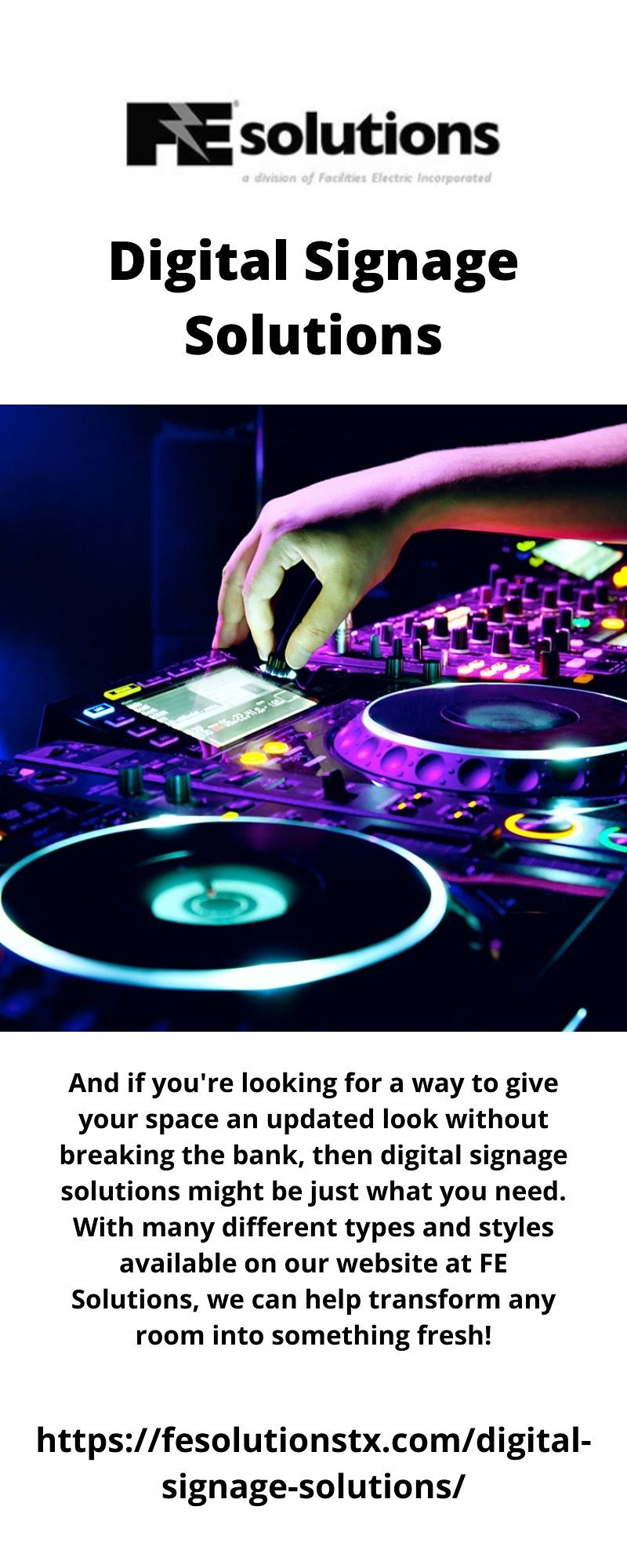The image is a screenshot of an advertisement set against a pure white background. The focal point of the ad is a title at the top that reads "FE Solutions" with a stylized lightning bolt separating the F and the E. Directly beneath, in bold text, it says "Digital Signage Solutions." The central portion features a square picture of a hand manipulating DJ equipment in a dark room illuminated by vibrant purple and blue lighting. Below the image, there is a substantial paragraph in black text. The paragraph explains, "If you're looking for a way to give your space an updated look without breaking the bank, then Digital Signage Solutions might be just what you need. With many different types and styles available on our website at FE Solutions, we can help transform any room into something fresh." Finally, at the bottom of the ad, a URL is provided: https://fesolutionsxdx.com.